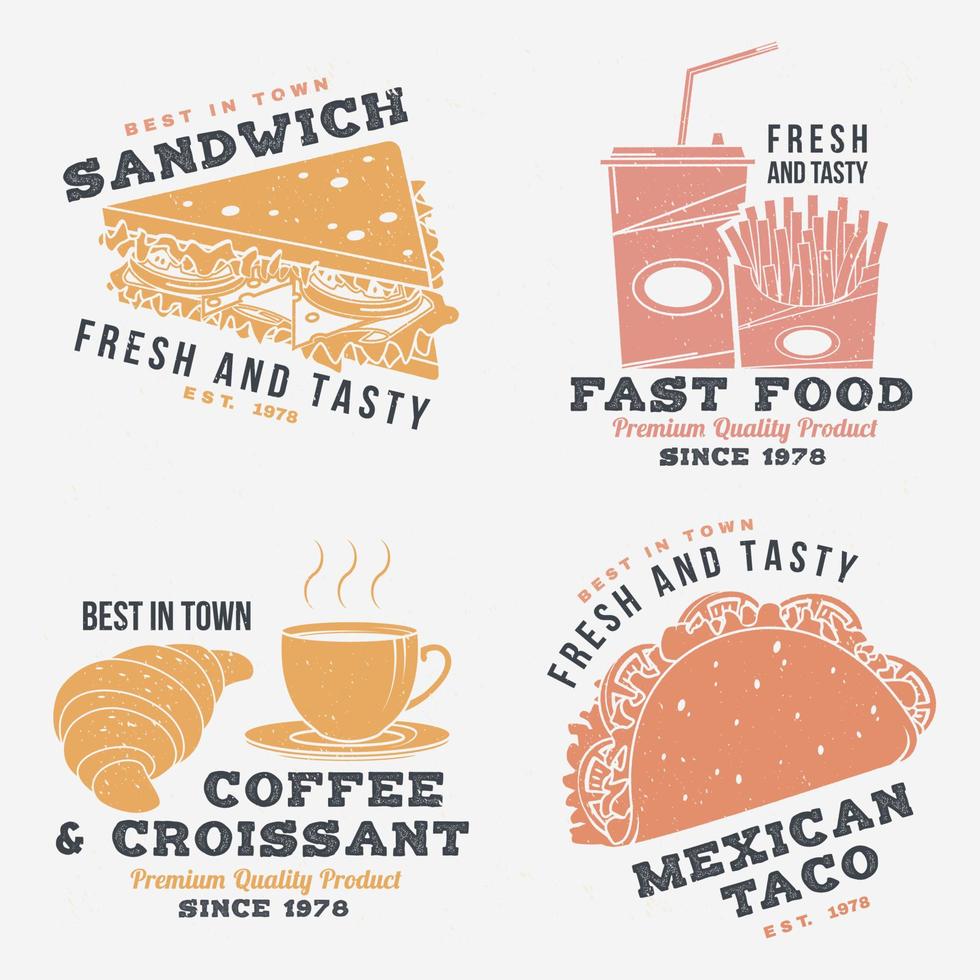The advertisement is a visually striking poster segmented into four distinct sections, each promoting different types of food offered by the same establishment. The poster, set against a white background, uses a consistent "fresh and tasty" theme across all sections, emphasizing the quality and appeal of the food. Each section also highlights the establishment’s long history since 1978.

In the top left, an orange-rendered image of a triangle-shaped club sandwich is accompanied by the caption, "Best in town sandwich, fresh and tasty." The top right features a red-shaded depiction of a drink with a straw and a container of upright-standing french fries, labeled "Fresh and tasty fast food, premium quality product since 1978." 

The bottom left corner showcases an orange image of a croissant and a cup of coffee, described as "Best in town coffee and croissant, premium quality product since 1978." Lastly, the bottom right corner displays a red illustration of a taco, adorned with the text "Best in town, fresh and tasty Mexican taco, established 1978."

The contrast between the red and orange sections and the cohesive nature of the captions suggest a versatile restaurant serving multiple types of cuisine, all promoting a high standard of "fresh and tasty" offerings.